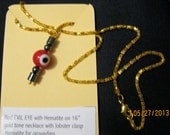This image features a gold-toned, 16-inch necklace with a lobster clasp, prominently adorned with a striking red evil eye pendant at the center. The eye, accentuated by a red bead detail and a central black dot, is surrounded by hematite beads, which are known for their grounding properties. The necklace is artfully positioned on a vertical yellow placard against a black cloth background. A white label at the bottom left details, "Red Evil Eye with Hematite on 16-inch gold-toned necklace with lobster clasp. Hematite for grounding." Additionally, a gold watermark dated "05-27-2013" is visible in the lower right corner. Despite the slightly blurry photograph, which affects the clarity of the chain and pendant, the distinct colors of gold, red, dark gray, black, yellow, and white are clearly outlined. The image appears to be styled for jewelry marketing purposes.